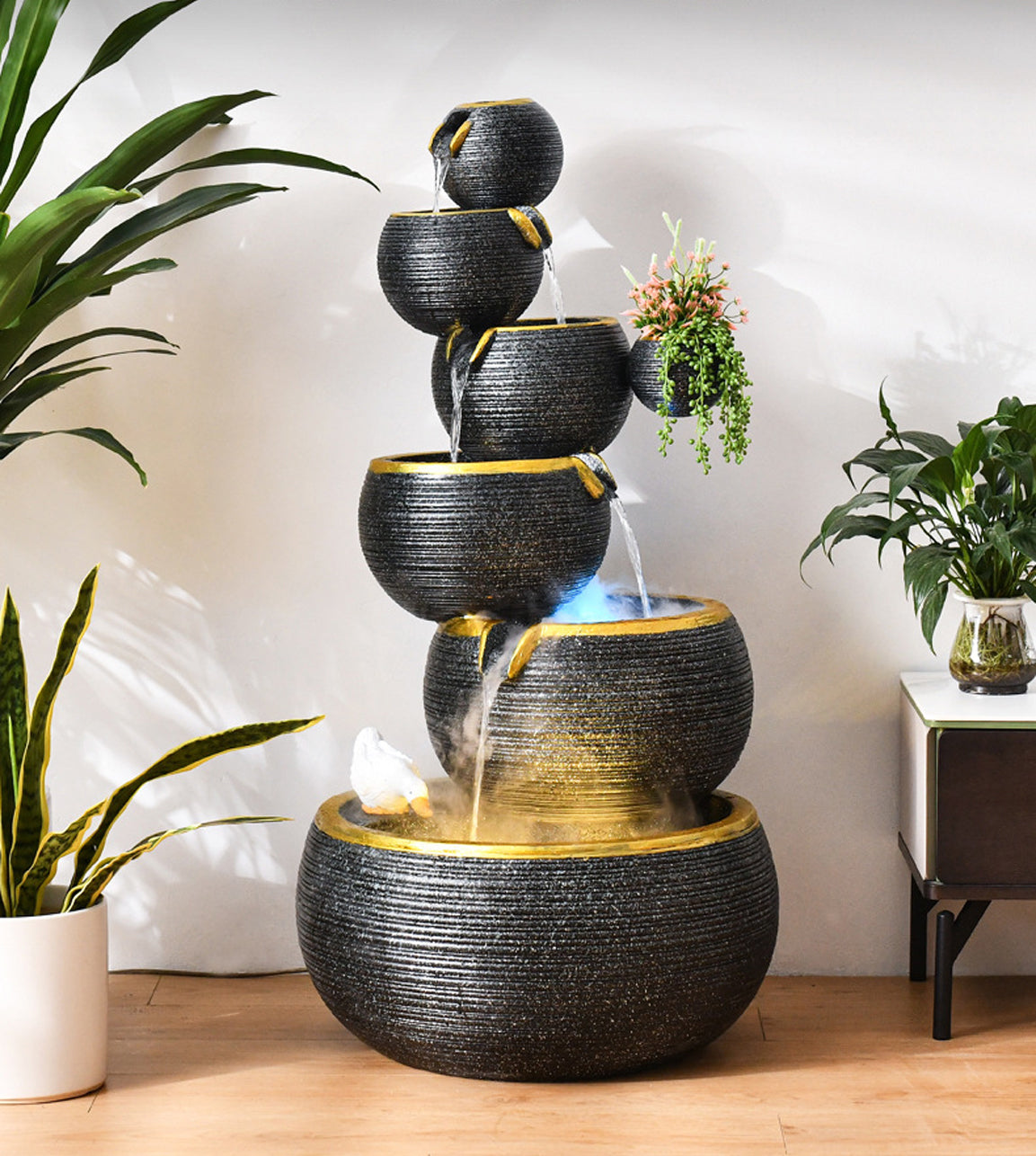This image showcases an intricate, tiered indoor fountain composed of six black bowls, each adorned with horizontal striations and rimmed with gold. The bowls are arranged in a staggered pattern, alternately positioned to the left and right as they ascend. Each bowl has spouts on the side, allowing water to cascade from one level to the next, creating a serene visual and auditory effect. Notably, a smaller bowl is attached to the third bowl from the top, holding trailing succulents and pink and white flowers. The fountain, centered in the photograph, sits on a light-colored wood or laminate floor against a white wall. To the left, there is a white pot containing a snake plant and possibly leaves from a corn plant. On the right, a black-legged table with a white top supports a ceramic vase with a lush peace lily. The detailed textures and play of water make the fountain a captivating focal point in this indoor setting.